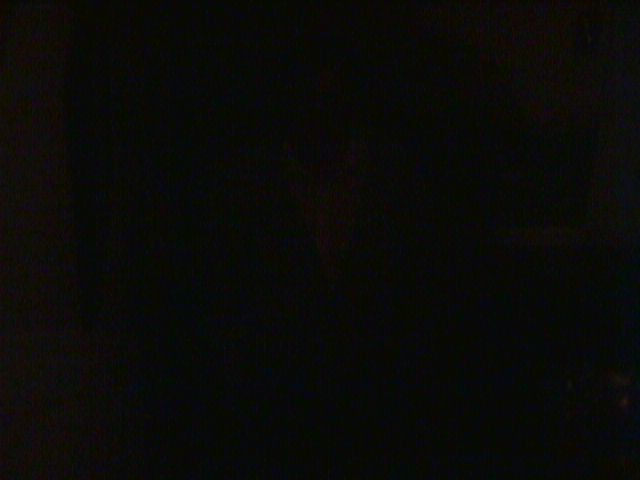This image depicts a matte black rectangle in landscape format, uniformly colored with no variations, shadows, or hues, creating an impression of pure, solid blackness. It resembles the shape of a four by six photograph and measures approximately one index finger length tall by two finger lengths wide, relative to an average woman's finger. While the majority of the image is pitch black, some subtle dark brown appears along the top right corner, forming a small heart. Overall, the image primarily consists of a deep, even black, making it difficult to discern any distinct imagery beyond the outlined detail.